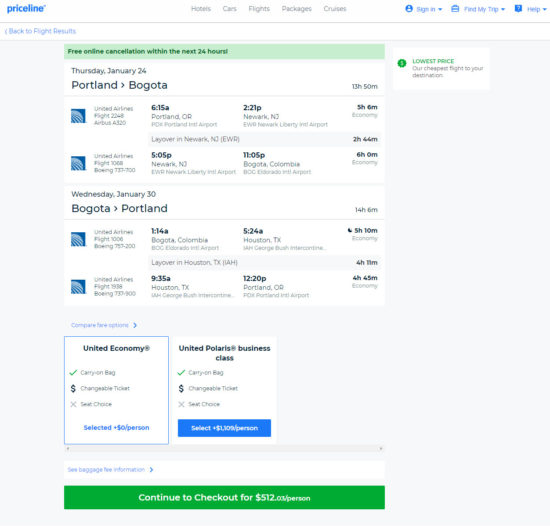The screenshot captures the top portion of a webpage from the Priceline website. In the upper left corner of the interface, there is a white rectangle featuring the "Priceline TM" branding in blue font. Immediately to the right of this, a navigation menu is displayed in gray font, listing various options like "Hotels," "Cars," "Flights," "Packages," and "Cruises." Further to the right, there are dropdown menus labeled "Sign In," "Find My Trip," and "Help."

Directly beneath this top section is another white rectangle with text in blue font that reads, "Back to Flight Results," accompanied by a left-pointing arrow.

The primary content of the webpage is framed within a large white square set against a light gray background. At the top of this white square, there is a light green bar with dark green text that states, "Free Online Cancellation within the next 24 hours." Below this, in black font, the text displays, "Thursday, January 24th, Portland to Bogota."

Following this, the page shows flight information that is unfortunately too small to discern. Below the flights are timetables detailing the journey. Midway down the white box, the text, "Wednesday, January 30th, Bogota back to Portland," is displayed. Additional timetables follow this information.

Lower sections of the white square include text in blue font, partially reading, "Compare Something," though it is too small to make out fully. Finally, towards the bottom, there are two outlined boxes labeled "United Economy" and "United Polaris Business Class."